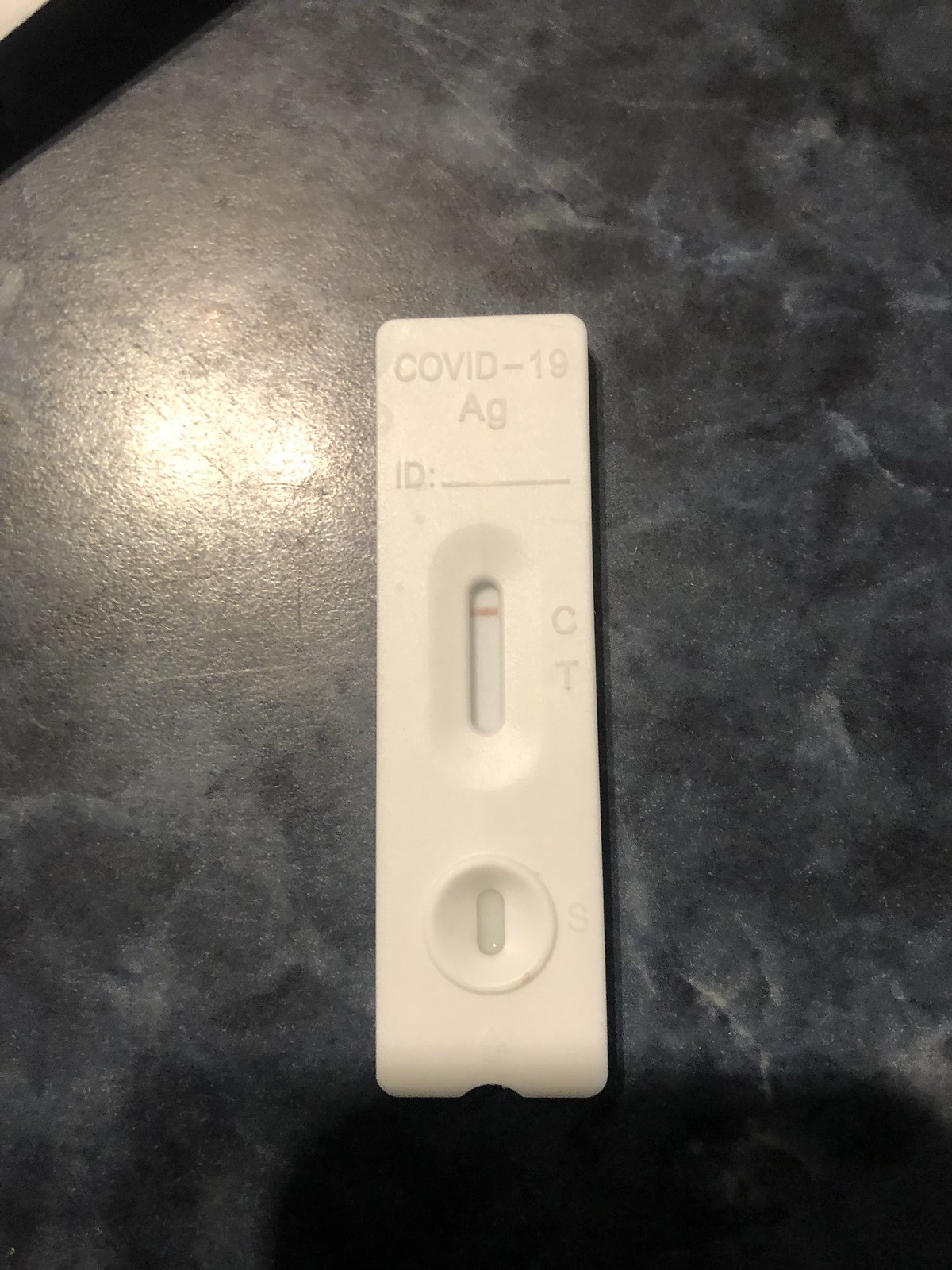The image showcases a black laminate countertop, designed to mimic the luxurious appearance of marble or granite. The background is predominantly dark with a noticeable shine in the upper left corner from an overhead light source, which adds a touch of elegance to the setting. A shadow is cast in the middle right section, providing a subtle contrast and depth to the composition.

Centrally positioned in the image is a white, vertically oriented rectangular object that captures immediate attention. At the top of this rectangle, the bold text "COVID-19" is prominently displayed, followed by "A-G" in capital letters. Below that, the label reads "ID" accompanied by a line, indicating this is a test kit. The central portion of the rectangle features an elongated oval viewing window, essential for reading the test results: one line indicates a negative result, while two lines would suggest a positive case.

Further down the rectangular test kit, there is a circular area with an opening designed for sample application. This is where the mixture from a cotton swab is deposited to facilitate the testing process. The precise labeling and strategic design elements underscore the object's purpose, making it an essential tool for COVID-19 diagnostics.